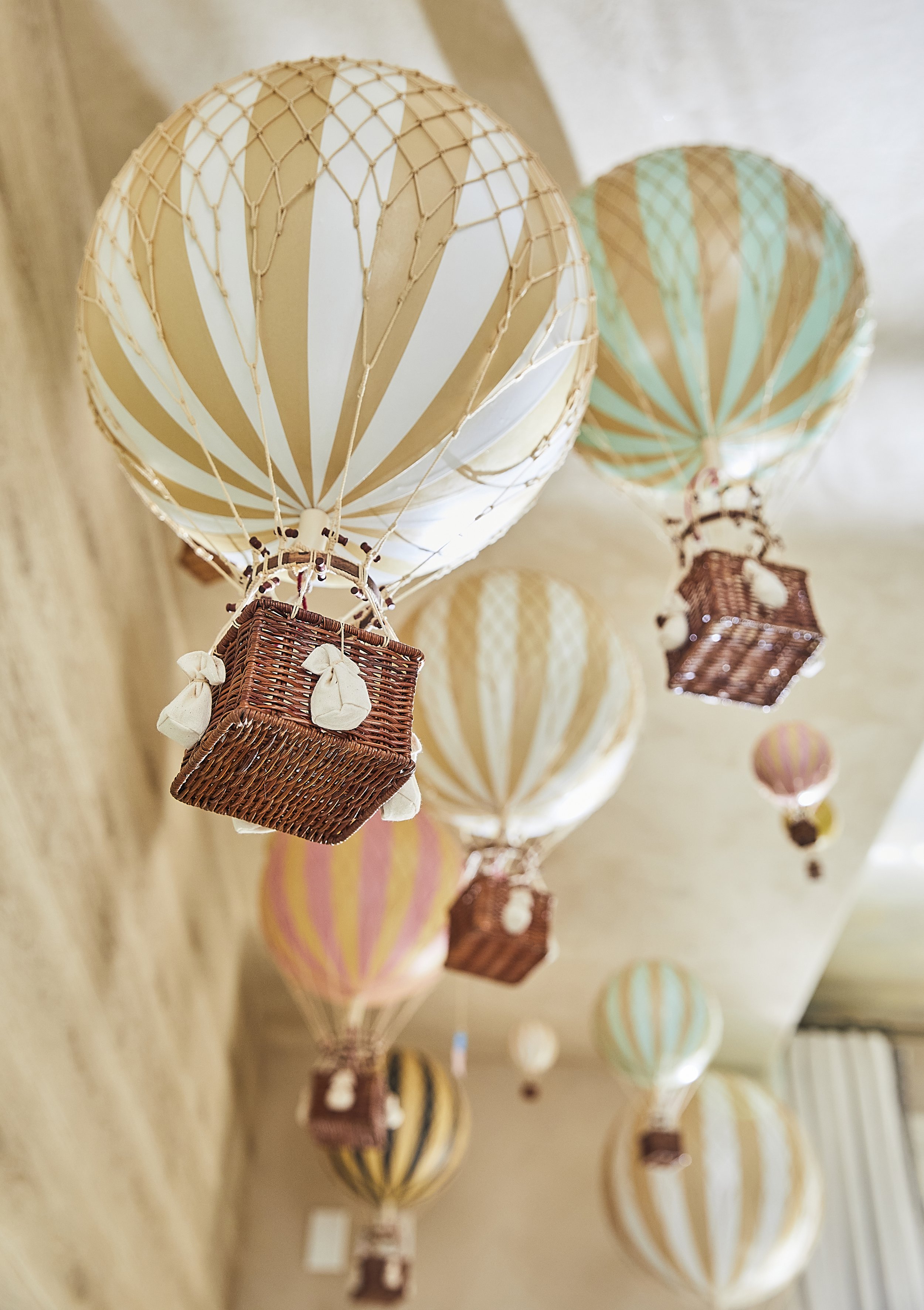The image depicts an indoor scene featuring a collection of miniature hot air balloon decorations suspended from the beige ceiling. The decorations are intricately detailed, each balloon having a small basket and sandbags attached, mimicking larger hot air balloons. The balloons feature various color patterns: some are white with gold stripes, others are green and gold, pink and gold, and black and gold striped. There's also a pink and peach balloon and a yellow with black striped balloon. Additionally, there are light blue or teal balloons with gold accents. The room has light tan walls and a glimpse of white curtains can be seen blurred in the background on the right side. The photograph captures the balloons from beneath, highlighting the whimsical view upward toward the ceiling. The muted coloring and slightly blurred background suggest a home setting, possibly showcasing crafted decor pieces.